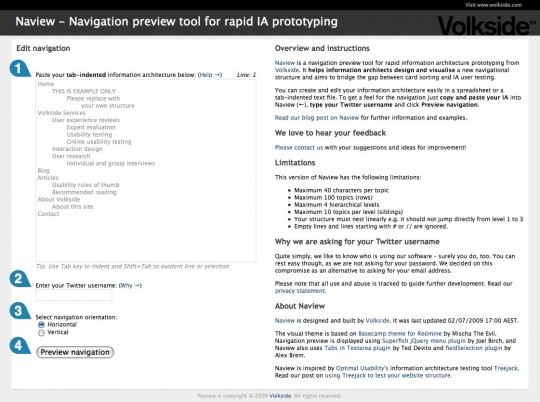The image displays the NavView Navigation Preview Tool, designed for rapid Information Architecture (IA) prototyping. At the top, there’s a title that reads "NavView Navigation Preview Tool for Rapid IA Prototyping" and a subtitle saying "Edit Navigation."

Highlighted in a blue bubble labeled "1" is the prompt to "Paste Your Tab Indented Information Architecture Below," followed by a placeholder text "Home. This is Example Only. Please Replace With Your Own Structure," and some illegible text beneath it.

Further instructions are listed below:

**2. Enter Your Twitter Username:** followed by a text box.

**3. Select Navigation Orientation:** with options for Horizontal and Vertical navigation orientation, where Horizontal is selected.

A blue box labeled "4" includes a button with "Preview Navigation."

On the right side of the image, under "Overview and Instruction," there is a description: "NavView is a Navigation Preview Tool for Rapid Information Architecture Prototyping. On the bulk's side, it helps Information Architects design and visualize a new stuffing structure."

Please note the typo "on Vulk's side." It should be corrected to "on the bulk's side" if referring to the larger part of the tool's functionality.